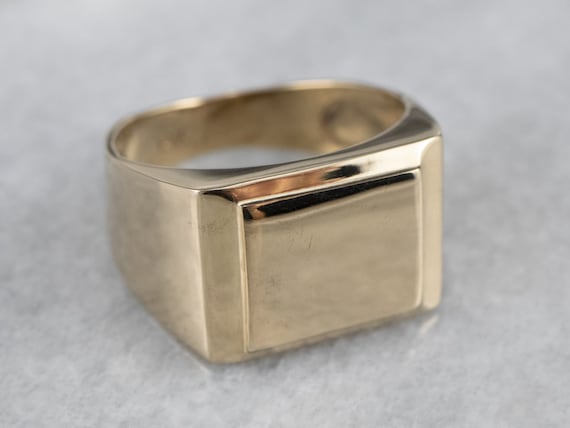The image depicts a large, chunky gold-colored ring, potentially made of real gold, lying on a marbled grey and white surface, possibly stone or granite. The ring itself is notable for its solid, square-shaped design on its top, which lacks any gemstones or prints. It features a flat square front that transitions smoothly from a wider to a narrower band as it encircles back to the other side. This square section, reminiscent of a high school graduation or sports championship ring, is also outlined by the side profiles of the ring which become the band. The ring is adorned with subtle imperfections and minor marks, suggesting it hasn’t been polished. A faint, distorted reflection of the photographer can be seen on the ring’s surface, adding a minor detail to the overall viewing experience.